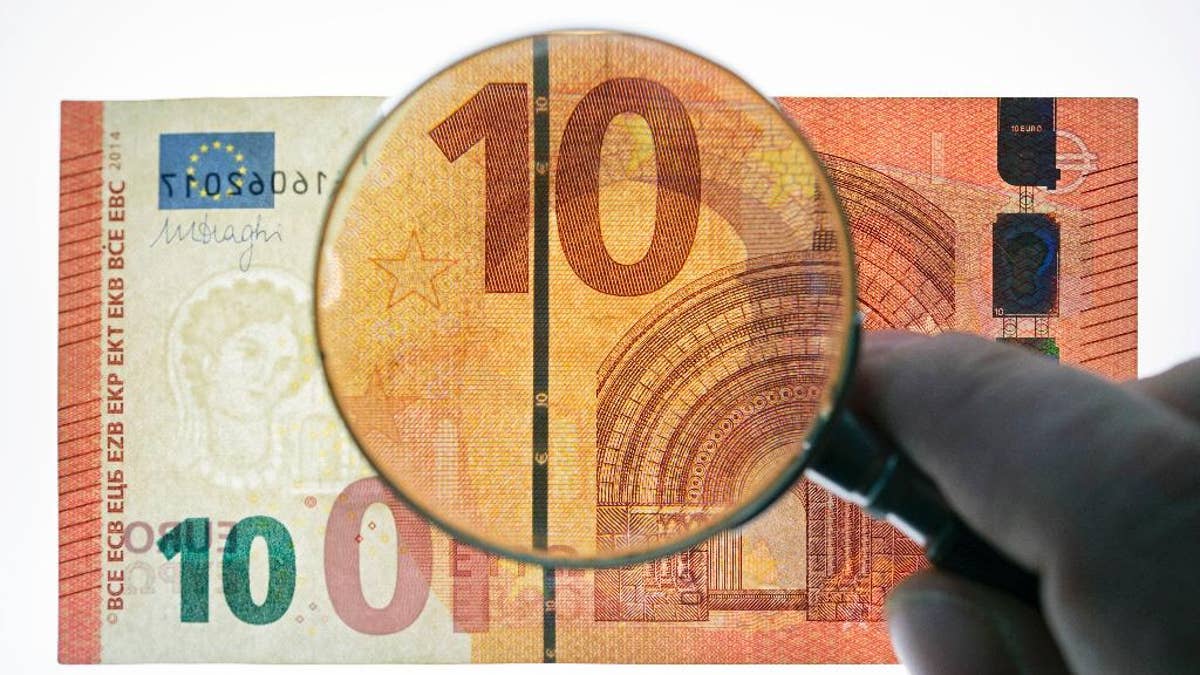This close-up image features a 10 euro banknote placed on a light table, illuminated to reveal intricate security elements. A hand, characterized by a gray glove, holds a magnifying glass over the center of the note, enlarging the intricate details. The banknote, primarily in coral and peach hues, showcases a green number 10 in the bottom left corner, which is prominently magnified. Surrounding the magnified area, the note displays a red reversed 01 and an architectural illustration of a stone arch in orangeish-red, symbolizing monumental European structures. 

On the far left, a vertical coral band features a sequence of multilingual abbreviations in different character systems, including BCE, ECB, and others, symbolizing the European Central Bank. Above this sequence is the European Union flag, depicting a circle of stars on a blue background. Additionally, the euro note is adorned with a watermark of a woman's head and a red outlined star, both visible through the translucent material. A series of blackish-blue squares, partially obscured by the holder's gloved finger, run along the right side. The overall composition highlights the sophisticated design and security features of the banknote, illuminated in vivid detail.